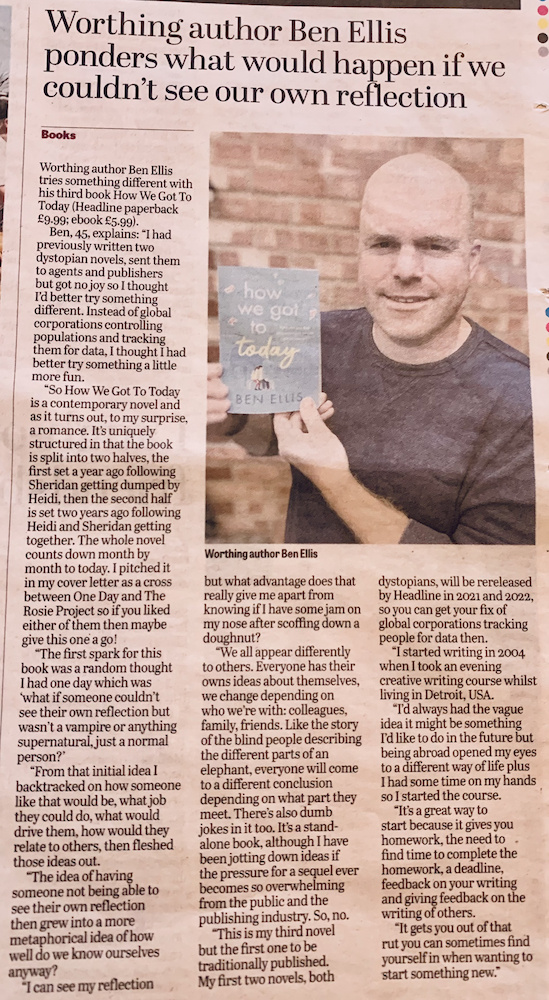In this detailed image, a newspaper article is printed on light purple paper, with the headline: "Worthing Author Ben Ellis Ponders What Would Have Happened If We Couldn't See Our Own Reflection." The section is labeled "Books" and delves into author Ben Ellis's latest literary endeavor. This is his third book, titled "How We Got to Today," in which he explores the intriguing concept of a world without personal reflections.

Accompanying the article is a photograph. In the background stands a prominent red building, while in the foreground is Ben Ellis himself—a bald man dressed in a black shirt. He holds up a blue piece of paper featuring the title of his book, "How We Got to Today," along with his name. The newspaper article spans three columns that surround Ellis's photo, indicating a substantial and in-depth coverage of his work and ideas.